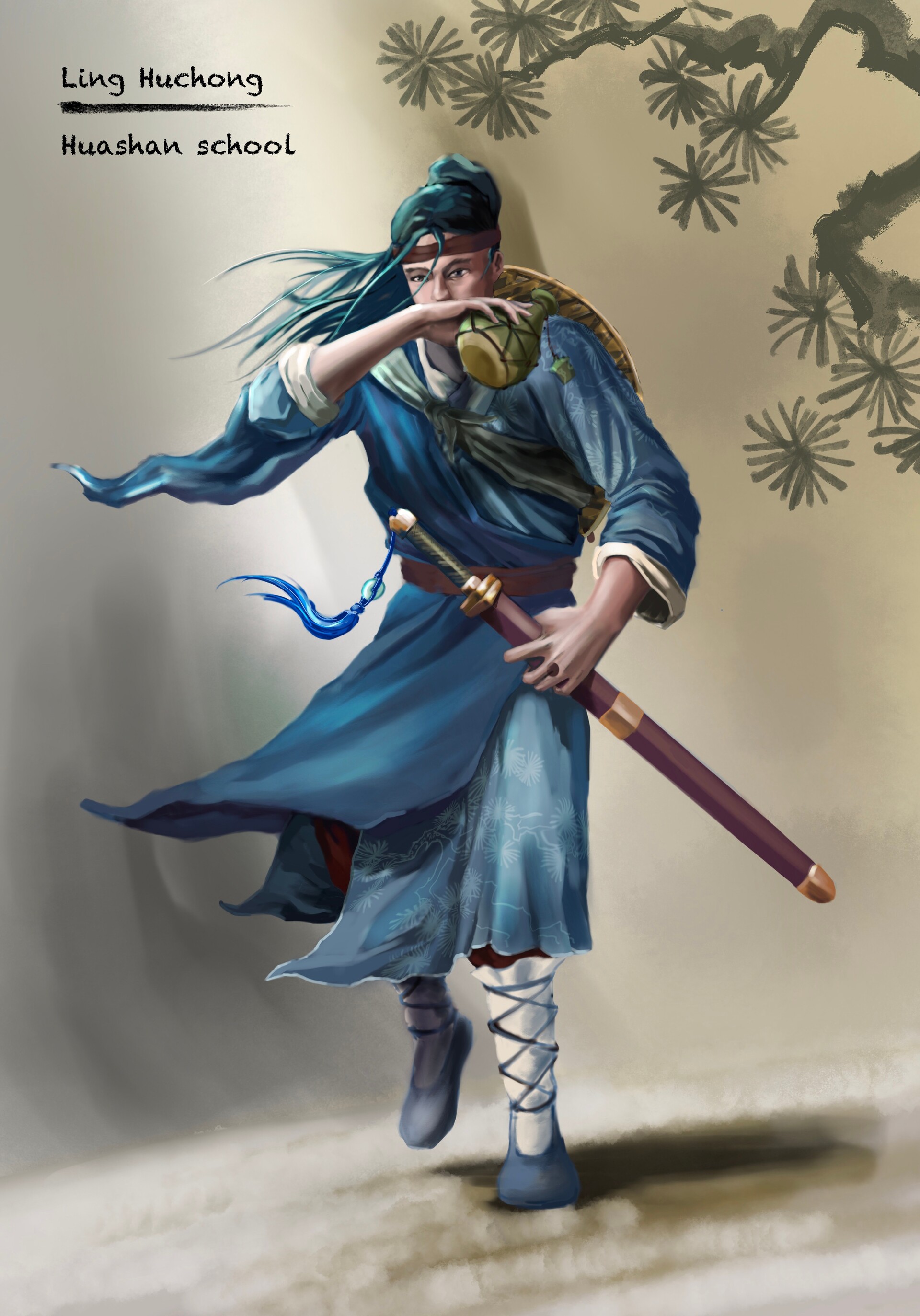The image is an Asian-style drawing featuring a central figure, presumably a warrior, depicted with great detail. The background is blurred and faded with grays and tans, and in the upper right corner is a silhouette-like tree with asterisk-shaped leaves or sprouts. The top left corner of the image includes black text that reads "Ling Huchong, Hua Shan School." 

At the center of the composition stands the main figure, defined by teal-colored, long, flowing hair tied up in a bun, which appears to be swept to the left by the wind. The figure has a red headband and is adorned in a flowing, dark blue robe secured with a red belt. They have a fair complexion and are holding a green vase or urn in their right hand, which is also wiping their lips just below their nose. 

Their left hand, positioned below the waist, grasps a brown scabbard with a gold band in the center, a gold tip at the bottom, and a gold band around the top where the sword is inserted. At the top of the sword, there is an attached feather that carries a blue hue. The figure's attire also includes old-style, lace-up shoes that tie up their calves. The overall scene suggests a moment of quiet reflection or readiness, emblematic of traditional Chinese artistry.